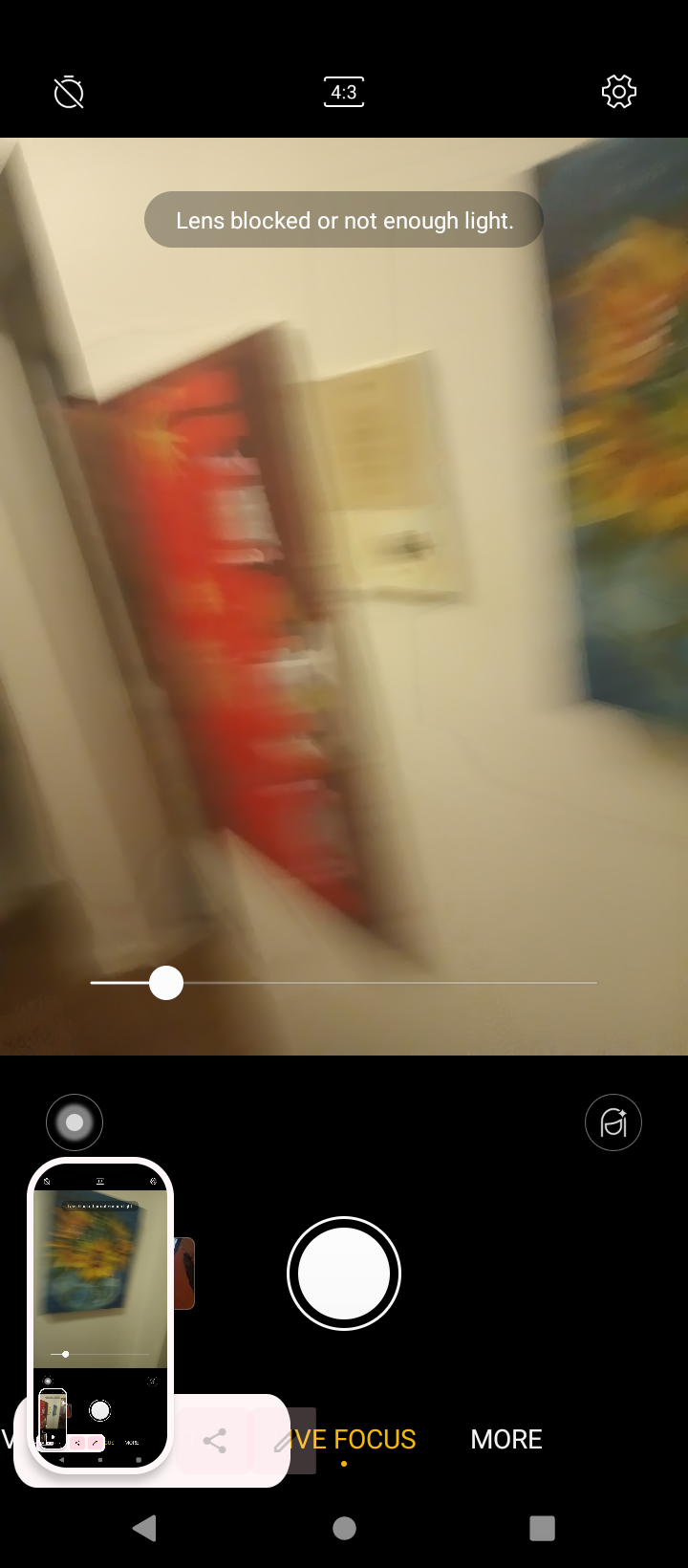The image is a blurry color photograph resembling a screenshot of a smartphone camera's display. The photo seems to have been captured accidentally while the person was walking, indicated by the motion blur and a warning message "lens blocked or not enough light" displayed on the screen. The upper portion of the screenshot features a black band with small white icons, including a circle with a line through it, the number "4.3", and a settings button. Below these icons, the camera display shows a blurred wall with two distinct pieces of artwork: a red painting in the center and to the right, a partially visible blue painting with yellow flowers. The screen's bottom third is occupied by a larger black band with various camera control icons, including a white circle (presumably the capture button), playback controls, and text stating "focus more." Overall, the image is a confusing blend of an in-motion photograph and a mobile camera interface, depicting an unfocused attempt to capture wall art.